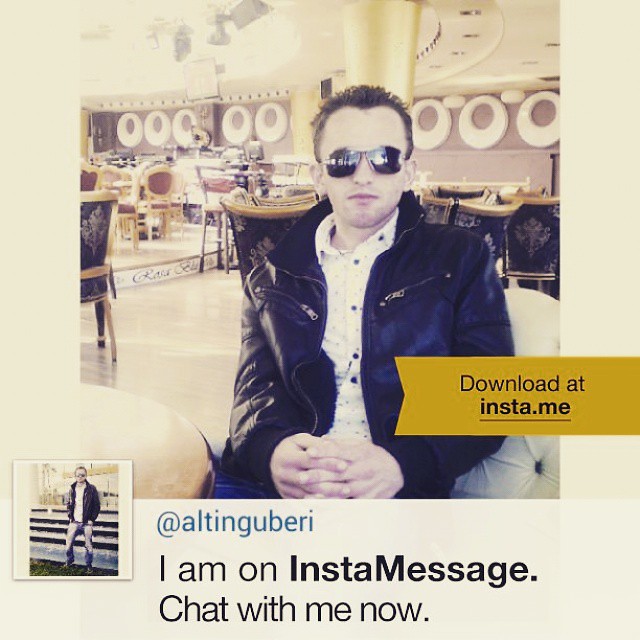The image appears to be a social media profile page, likely from an Instagram message account. Featured prominently in the center-right is a young man with short spiky brown hair, wearing sunglasses, a black leather jacket, a white shirt, and jeans. His hands are folded in front of him. The background suggests a restaurant setting, with chairs and tables evident; some chairs are adorned with black and gold, while others on the left have splashes of gold and red. A large golden beam is notably present behind him.

Below the main image, which is set against a white background, there is text that reads "@Altinguberry" with the phrase "I am on Insta message. Chat with me now." Additionally, a gold banner across the picture displays the URL "download at insta.me," which is underlined. On the bottom left, there is a smaller inset image of the same man standing against a fence, facing slightly to the left. Circular patterns are noticeable on the wall in the background of the main image, contributing to the restaurant ambiance.